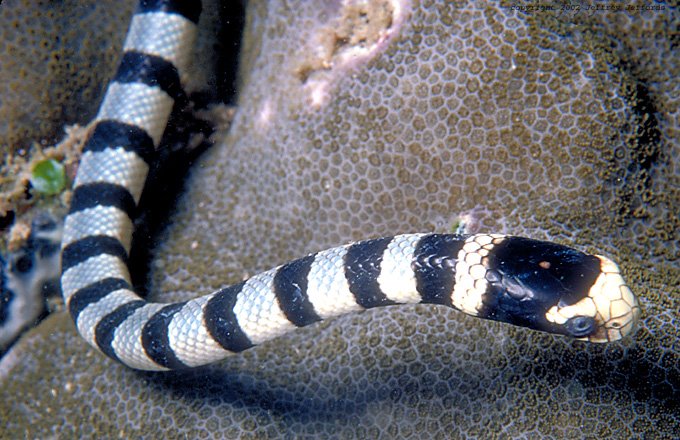The image features a detailed, close-up, top-down view of a banded snake with distinct white and black stripes, with the very front of its head being white and the top mostly black. Its eye is open, and it appears to be in motion, looking to the right. The background suggests an aquatic environment, implied by a bluish tint and a possible watery surface, overlaid with hexagonal or circular textures that resemble coral. This surface is brown with light blue hues and has slightly raised circular ridges that could trigger trypophobia. Additionally, some green vegetation, possibly a clover, is visible towards the left side of the image. The tail of the snake is out of frame, emphasizing its length as it moves across this textured, possibly aquatic setting.